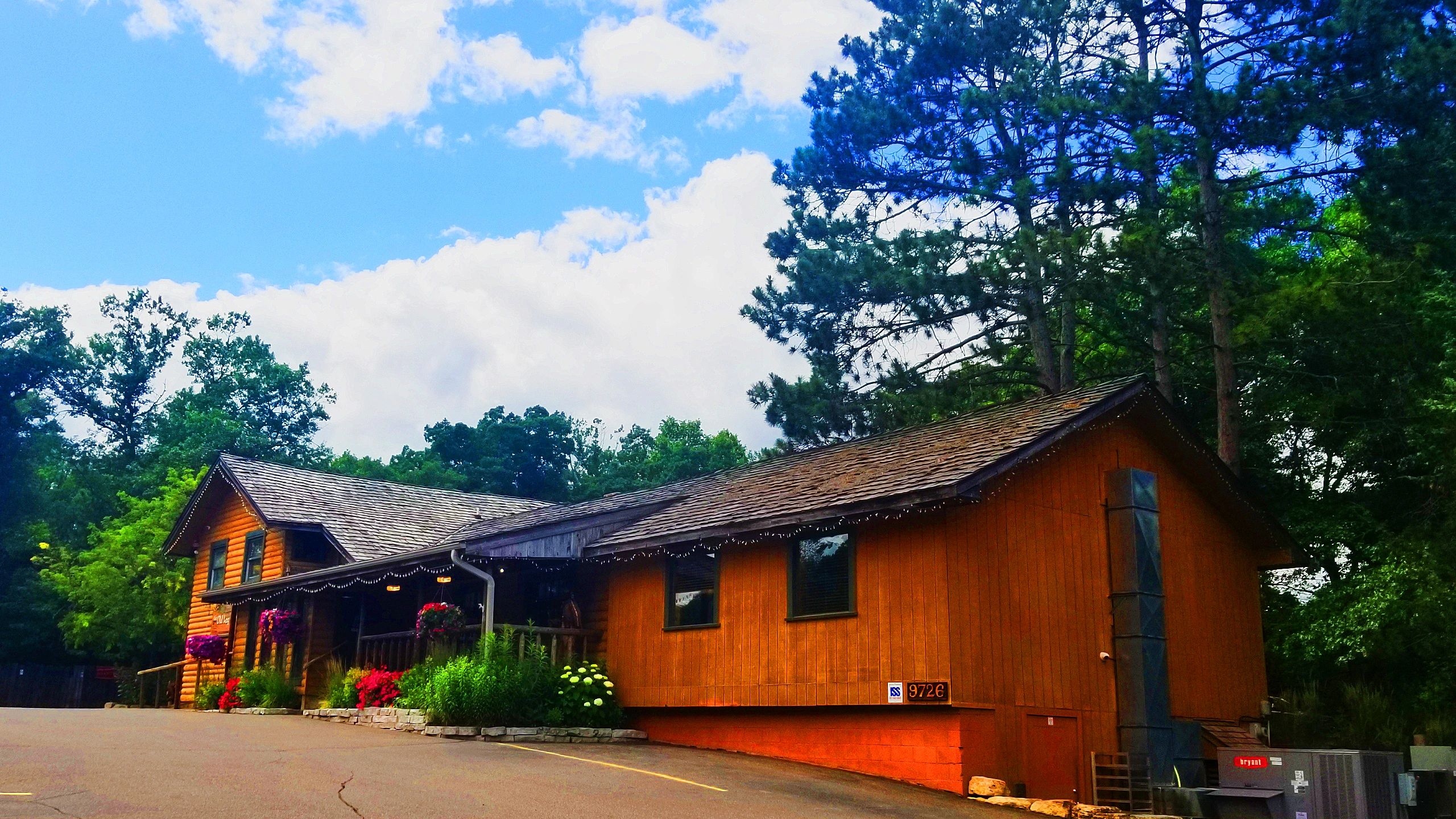The photograph depicts a charming single-story, brown wooden house situated on a sloped terrain, with a mix of vertical and horizontal wooden boards on its exterior. The house, identified by its street number 9726, boasts a blackish-blue roof adorned with some pine debris. The scene is lit by natural light under a partly cloudy sky. 

In the foreground, there's a covered porch surrounded by a vibrant wraparound garden bed, teeming with various green and flowering plants. Pots of hanging flowers further embellish the porch. To the lower right stands a metallic air conditioner unit, presumably contributing to the home's comfort. 

Trees provide a lush green backdrop on the left and center left of the image, contributing to the serene outdoor ambiance. Additional elements include a possible generator and hints of a roadway or parking spots in front. The house, which might also be a farmhouse or a restaurant, presents a welcoming front with visible windows and a cozy, flower-rich porch area.